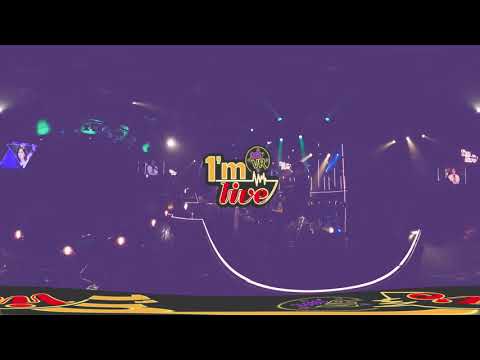The image appears to capture a dimly lit concert or bar scene, shrouded in a purplish hue that makes details challenging to discern. Central to the image is a stage featuring performers, possibly a band or a solo act, with lights of various colors—including green, yellow, red, white, and blue—spread sporadically throughout the scene. On the left side of the image, there is a large TV screen displaying the text "1M live" in bold, colorful letters: "1M" in yellow with a white outline, and "live" in red. The term "VR" appears in black and gold in the upper right corner. The rectangular image, framed by a black header and footer, suggests a unique stage design. The setting hints at an intimate venue, perhaps reminiscent of a romantic, coffee-shop-like environment.